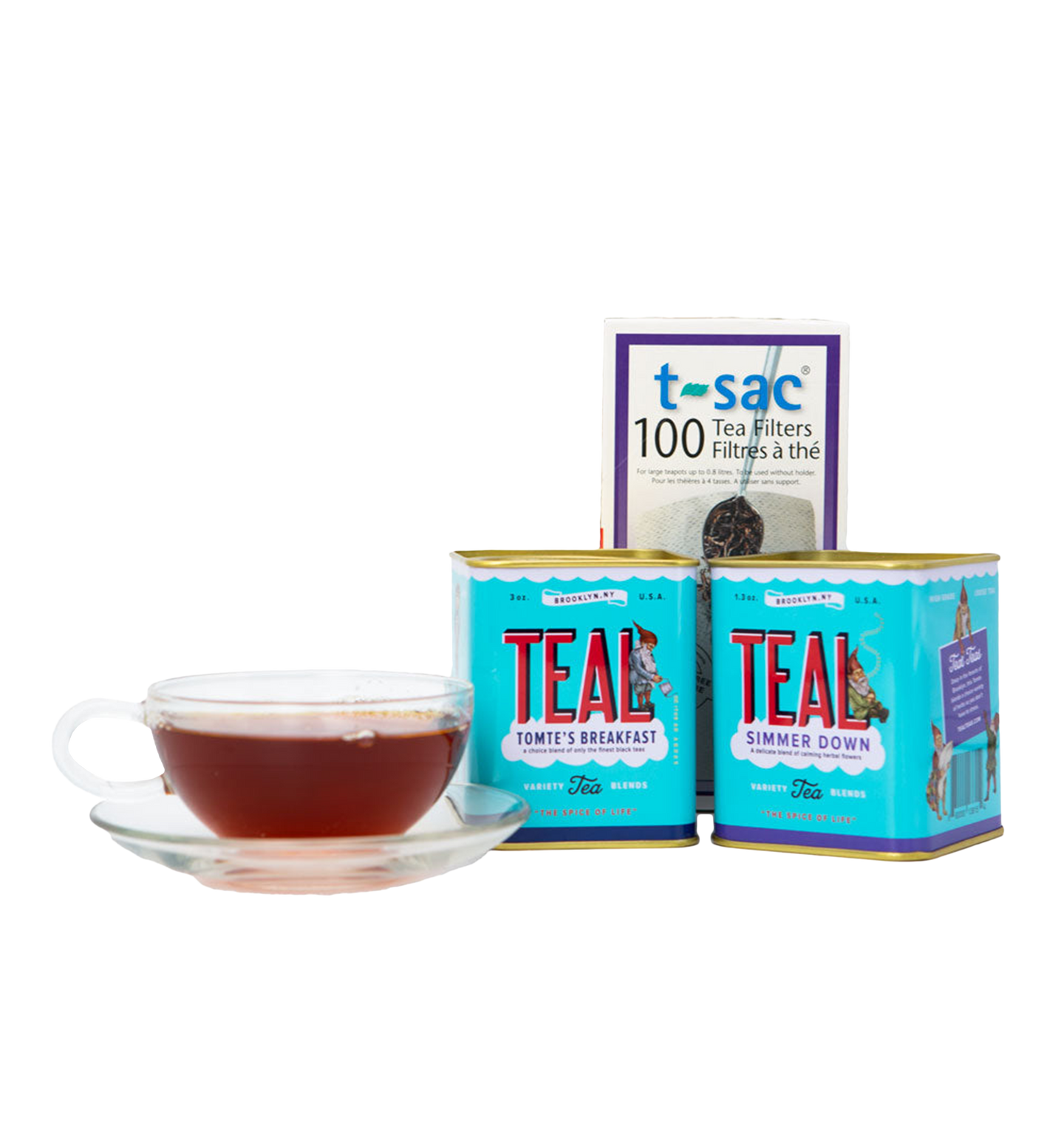This detailed image shows an advertisement for Tom’s Breakfast Teal Tea, featuring two prominently displayed square blue tins labeled "Tom T's Breakfast" and "Simmer Down." To the left of these tins is a clear cup containing brown tea, resting on a matching clear saucer. Above the tins is a white paper container labeled "T-SAC, 100 tea filters," with additional foreign language text and an image of a spoonful of tea, positioning the tea products centrally within the composition. The vibrant design on the tea tins, characterized by a mix of red, purple, black, and white text on a striking teal background, makes the packaging visually appealing. Despite the less attractive tea filters packaging, the overall presentation is enticing and expertly crafted to draw attention.